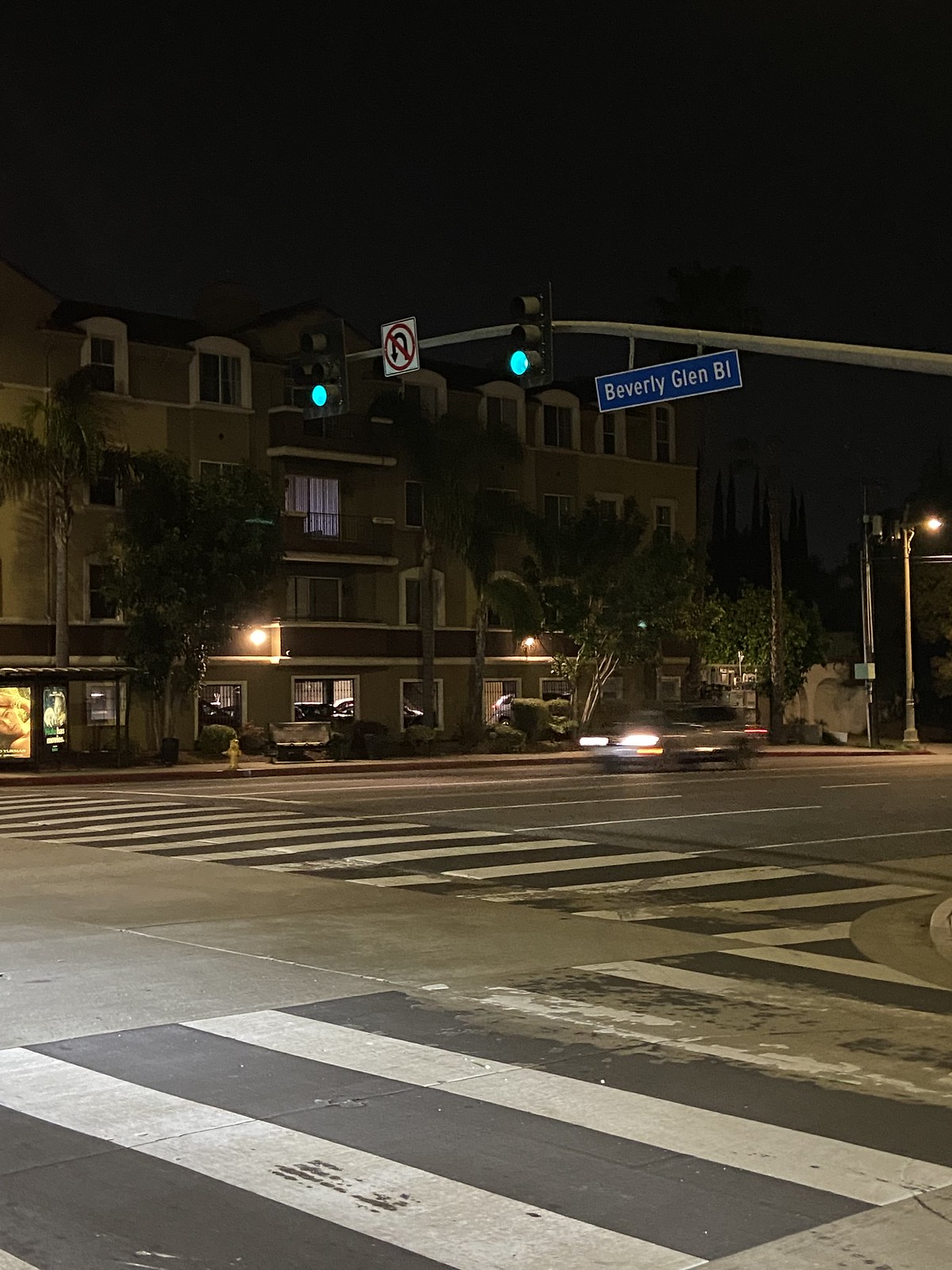A nighttime photograph captures a city intersection under a pitch-black sky devoid of stars due to light pollution. The intersection features two prominent zebra crossings: one stretches diagonally from the bottom left corner to a point about a third of the way up on the right-hand side, where the curved edge of a sidewalk is visible. The second zebra crossing extends from this point towards the central left side of the image. The pale gray road surface is marked with clearly painted lanes.

A single vehicle travels from right to left along the road. In the background, street lights illuminate the scene, and a yellow-painted fire hydrant stands out. The buildings lining the street appear to house storefronts on the ground floor; the structures are brown with dark brown or black awnings. One building has lights on in the upper floors, indicating potential residential spaces.

Dominating the top third of the image, a traffic light pole extends from right to left, supporting two green traffic lights. A 'No U-turn' sign, featuring a red circle on a white background with a crossed-out U-turn symbol, is positioned between the lights. A blue street name sign attached to the pole reads "Beverly Glen Boulevard."

This detailed scene combines urban elements—pedestrian crossings, vehicles, storefronts, and traffic signals—against a backdrop of a starless city sky.